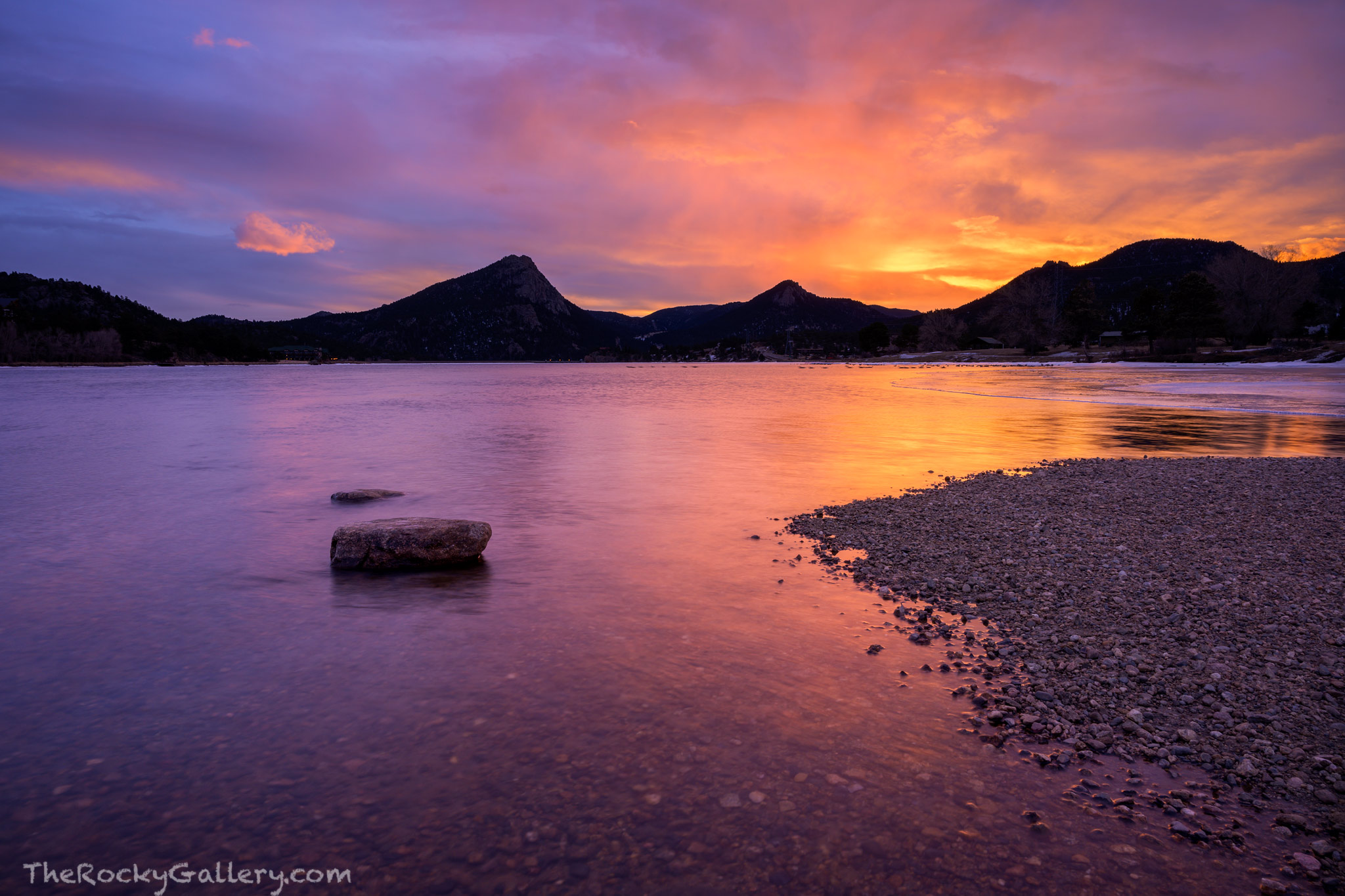This stunning outdoor photo captures a serene sunset scene with text reading "therockygallery.com" in the bottom left corner. The horizon is dominated by a silhouette of dark mountains, backlit by the setting sun, which casts a gradient of colors across the sky, seamlessly transitioning from yellow to orange, then to pinkish hues, and finally into blues and purples as it darkens. Below the mountains, a tranquil lake mirrors these vivid colors, its surface so calm it resembles glass. In the foreground, the shallow water reveals tiny pebbles, and a prominent flat-topped rock emerges from the water. To the far right, a small rocky shoreline edges into the scene, adding depth and texture to this breathtaking landscape.